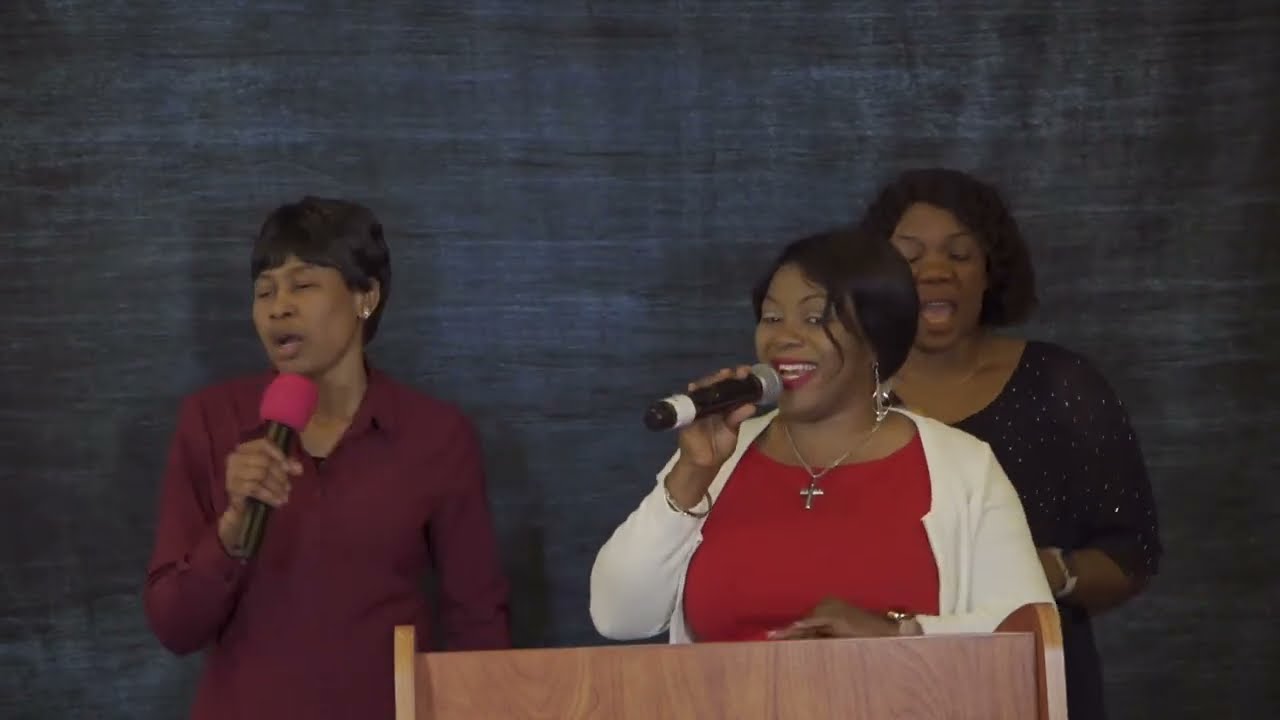The image depicts a poorly lit but full-color, horizontally rectangular photograph, possibly a screenshot from a video taken indoors. It features three African-American women who appear to be singing, likely in a church or performance setting, as suggested by the presence of a crucifix necklace worn by the woman front and center. The background is a plain, dark blue curtain with visible shadows, emphasizing the light source directed at the subjects. The woman to the left wears a purple, long-sleeved shirt and sings with her eyes closed, holding a microphone with a reddish-pink top. The central woman stands behind a brown podium, dressed in a red shirt, white sweater, and a crucifix necklace, holding a microphone in her right hand. To the right and slightly behind, the third woman is seen in a sparkly blue top, possibly a dress, though it's uncertain if she holds a microphone. Together, the trio is captured mid-performance, their open mouths indicative of singing against the indistinct, shadowed backdrop.